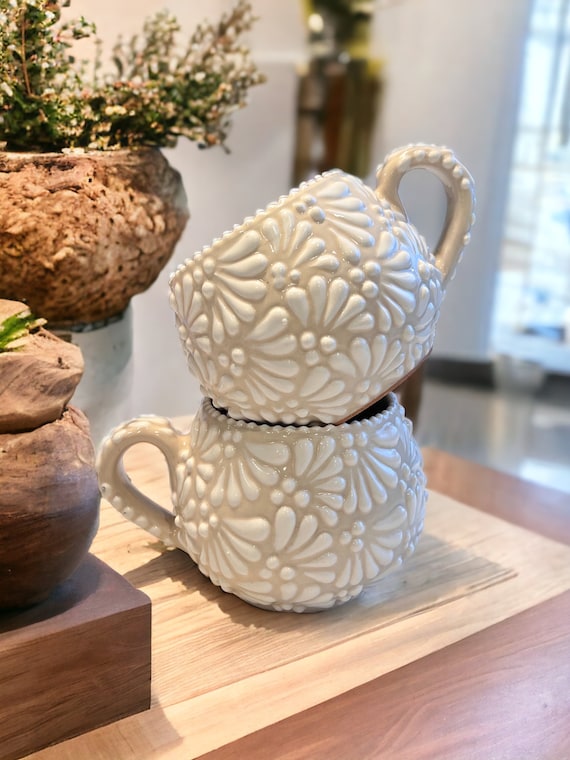In this beautifully aesthetic photo, the focal point is two ornately decorated coffee mugs stacked on a wooden table. The mugs, both a pale tan or beige color, feature an intricate raised floral pattern in white, including three berry-like dots and leaf-shaped designs extending from the berries. One mug sits directly on the table while the other is tilted at a slight angle on top of it. Surrounding the mugs on the tabletop are various wooden decorations, and in the background, there's a wooden stand accompanied by a pot with green foliage. The warm tones of the wood and the delicate details of the mugs create a pleasing visual, reminiscent of carefully curated social media photography.